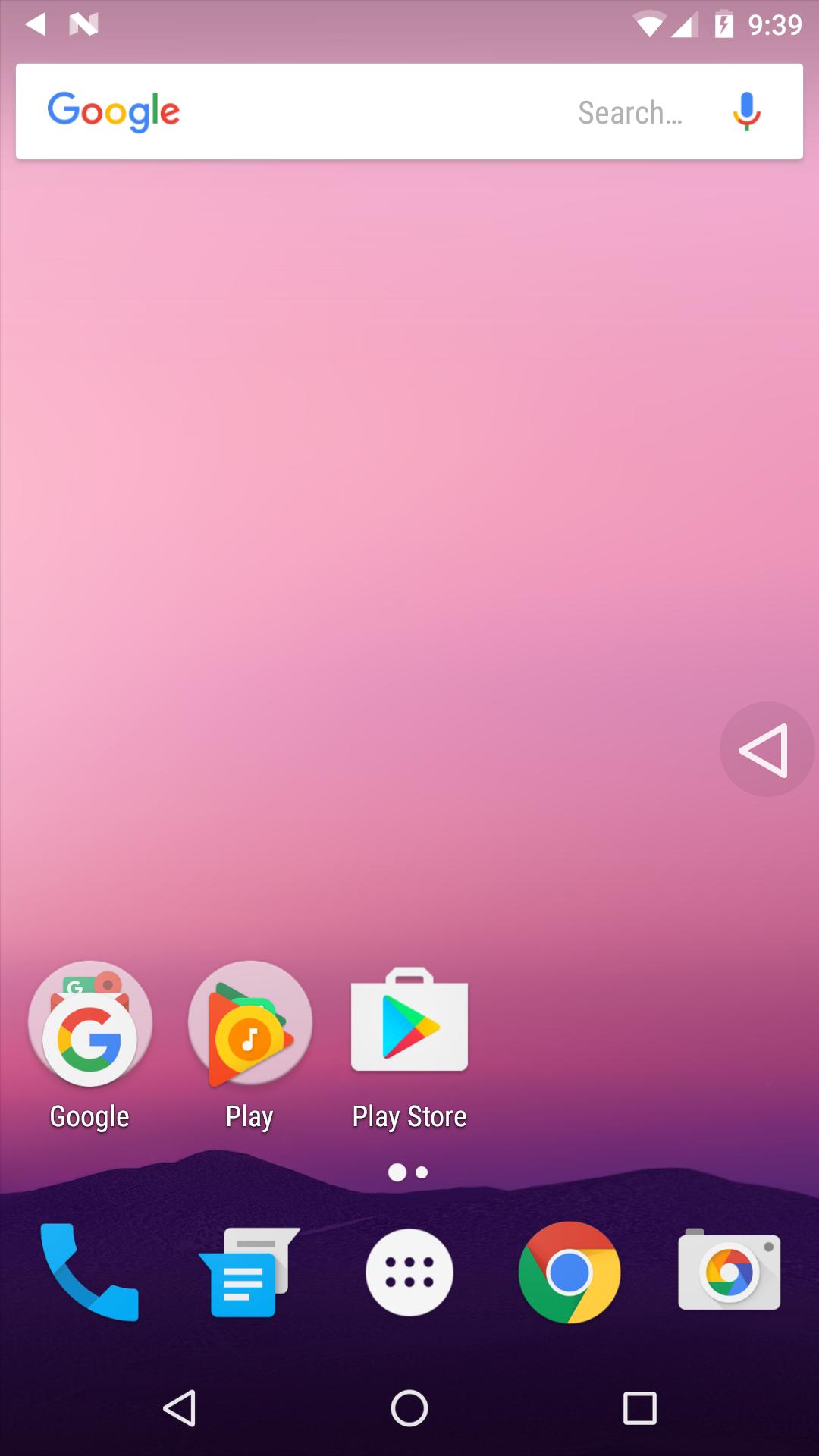This is a detailed description of a smartphone screen. At the top, it displays a notification bar with a "N" and a left arrow symbol, indicating a notification or navigation option. The status icons show an active Wi-Fi connection, cellular signal strength, and a battery charge level of 93%.

Centering the screen is a white Google search bar. The Google logo is prominently displayed in its characteristic colors: blue, red, yellow, blue, green, and red. Next to the search bar is a microphone icon for voice search functionality.

The wallpaper is an artistic depiction of a mountainous landscape in silhouette. The mountains at the bottom are a deep, rich purple transitioning to a vibrant pink sky above, which gradually lightens to a soft pink at the top.

Overlaying the sky are several app icons, including Google and the Play Store. Near the bottom of the screen, there is a row of navigational icons. These include a blue phone icon, a blue and white chat icon, and a circular button with six dots arranged in two rows and three columns, indicating app drawer access. 

Additionally, there is a Google Lens search button with a rounded outline in red, yellow, and green, housing a blue dot in its center. The camera icon also features Google's signature colors arranged in a circular pattern. 

This description provides a vivid snapshot of the screen, capturing both functionality and aesthetic elements.